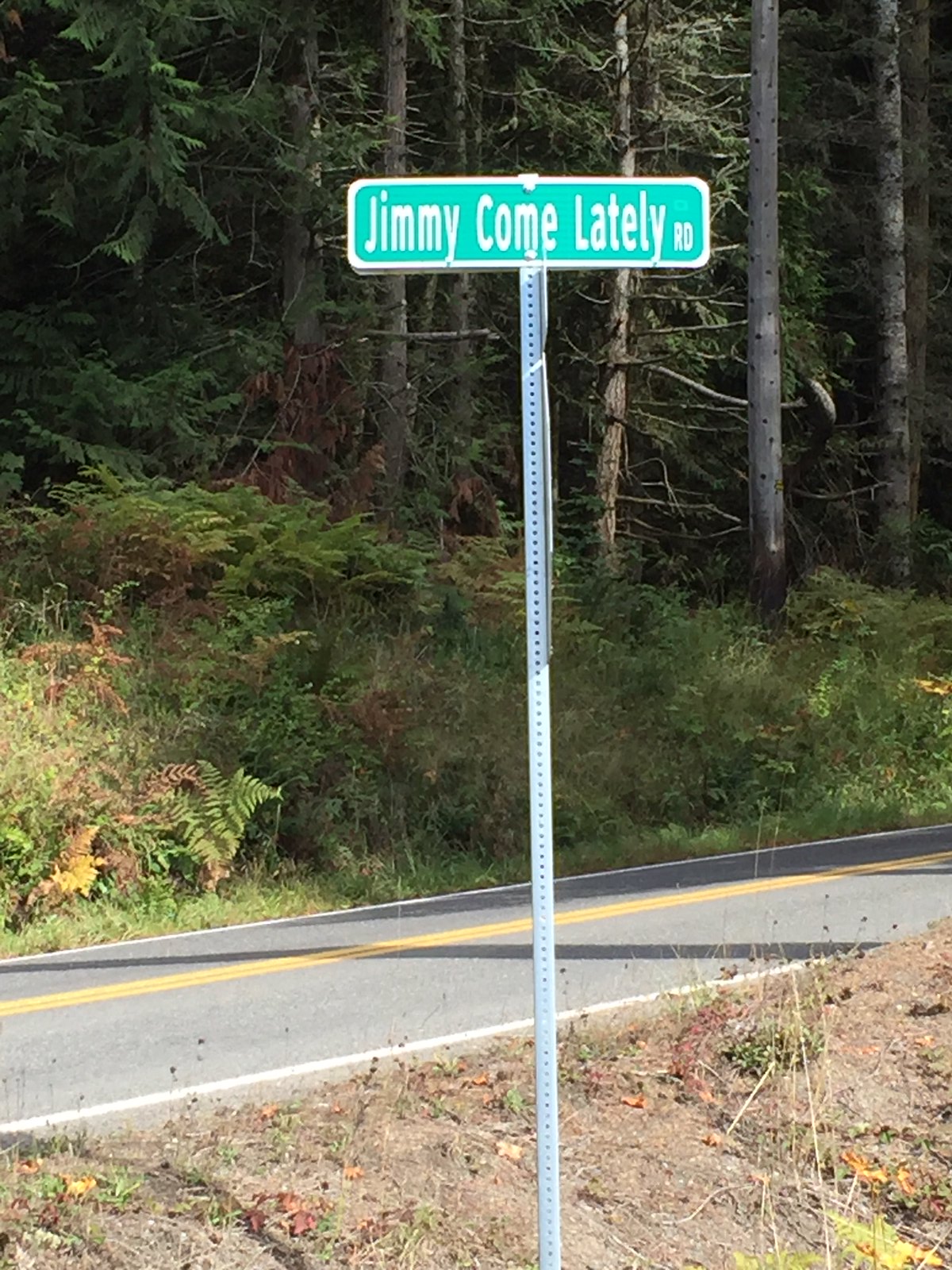A narrow two-lane road, aptly named "Jimmy Come Lately Road," stretches into an unknown distance. The road is devoid of vehicles and marked with a solitary yellow centerline. On the left side of the road, the ground is mainly bare, featuring patches of dirt interspersed with sparse, dried vegetation and fallen leaves. On the right side, a dense cluster of trees, grass, and weeds serves as a natural boundary, suggesting the edge of a forest that appears unmaintained and wild. A street sign, green with white lettering, stands prominently at the roadside, clearly identifying the name of this seemingly isolated path. The scene captures the quiet, untouched essence of nature meeting a solitary strip of pavement, inviting curiosity about the journey ahead.